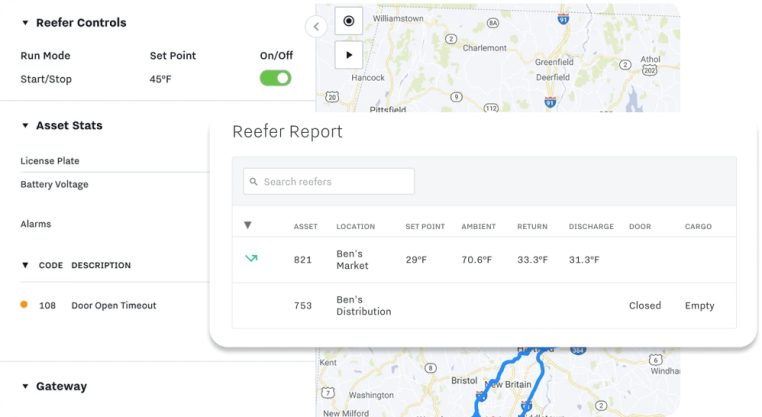**Caption:**

The page prominently features a map labeled "Reefer Controls," indicating a focus on refrigeration systems, possibly for transport. Detailed geographic markers such as Bristol and New Britain suggest the map depicts a region in the United Kingdom, with noticeable rivers at the bottom. On the left side of the page, the heading "Reefer Controls" is bold and slightly larger than the rest of the text. Below this heading, the section lists various operational modes: “Run Mode,” “Start,” “Stop,” “Set Point” (set at 45 degrees Fahrenheit), and options for "On or Off."

Further down, a bolder but smaller header reads "Assets," followed by entries for "Stats," "License Plate," "Battery Voltage," and "Alarms." Underneath this section is "Code Description," distinguished by a less bold typeface. This part details a specific code: "108," accompanied by a small orange circle. The description for code 108 is "Door Open Timeout."

Lastly, the bottom of the page features the bolded word "Gateway," with an arrow pointing downward, suggesting a link to additional information or another section.